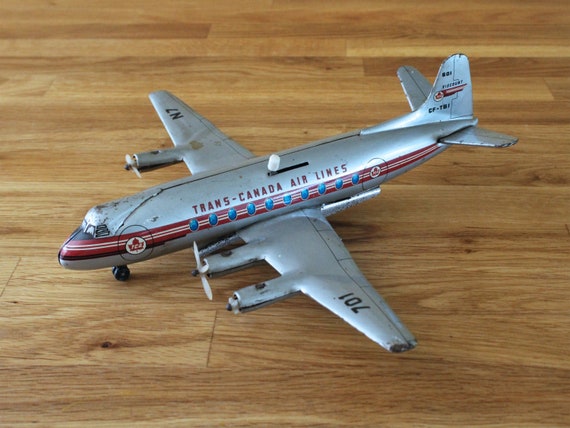The image showcases a vintage toy or model airplane made of a silvery gray metal with detailed red, white, blue, and black markings. The plane, adorned with a red and white stripe running from the nose to the rear, bears the label "Trans-Canada Airlines" prominently above blue oval windows along the side. A red maple leaf, indicative of Canadian identity, is encased in a white circle near the nose. The wings are marked with the numbers "701" on the left and "N7" on the right in black stenciled font. The airplane, positioned at a slight angle with its nose pointing to the lower left, is resting on a light brown wooden surface. Notably, the plane shows signs of wear, including some scuff marks and a potentially tarnished front, suggesting it's a well-loved vintage piece. A metal lever or switch is visible on the top, hinting at a functional feature, as well as an additional undetermined protuberance on the left wing. The overall atmosphere of the photograph is slightly overexposed with overcast lighting, emphasizing the nostalgic aura of the scene.